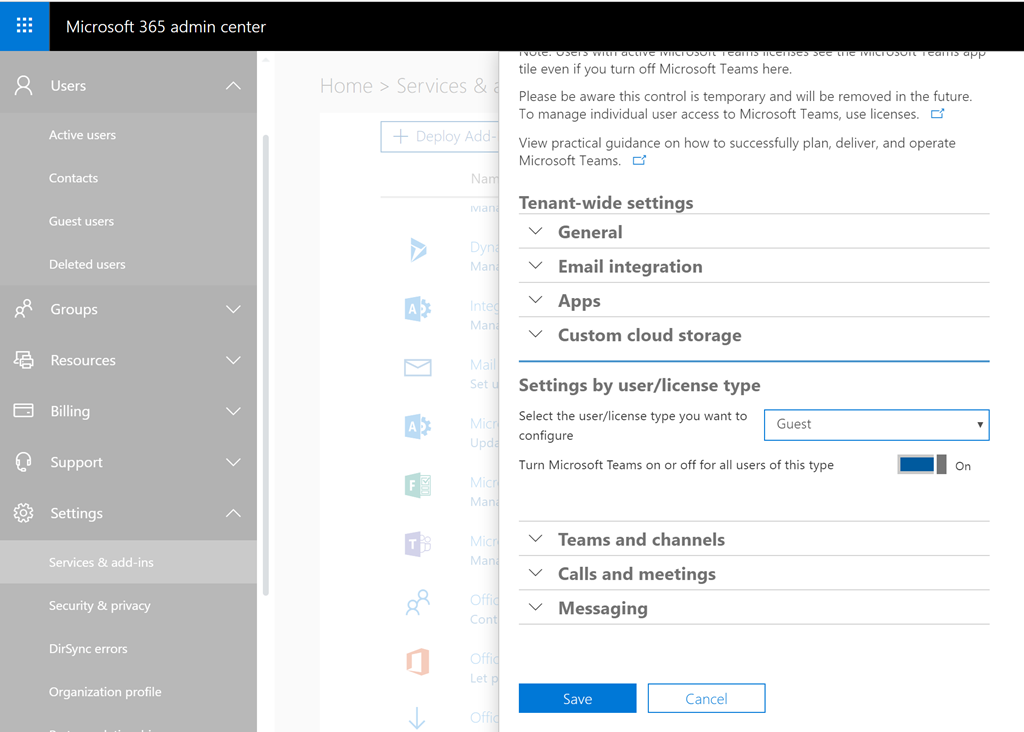**Detailed Caption:**

Screenshot of the Microsoft 365 Administration Center. The interface features a black rectangular bar at the top with the title "Microsoft 365 Administration Center." The left sidebar is set against a gray background and includes various navigation options: 

1. **Users**: Represented by an icon of people, with subcategories including:
   - Active users
   - Contacts
   - Guest users
   - Deleted users

2. **Groups**
3. **Resources**
4. **Billing**
5. **Support**
6. **Settings**
7. **Services & Add-ins**
8. **Security & Privacy**
9. **Directory Sync Errors**
10. **Organizational Profile**

To the right, a prominent notification informs users that a particular control is temporary and will be removed in the future. There is also practical guidance available on how to successfully plan, deliver, and operate Microsoft Teams. Further down, tenant-wide settings are displayed for "General," "Email integration," "Apps," and "Custom cloud storage." Settings by user and licensing type show options for "Guest" users, including sub-settings for "Teams and channels," "Calls and meetings," and "Messaging."

The main content area has a black background, with a highlighted blue box containing guest settings. At the bottom of the interface, two action buttons are present:
- A "Cancel" button with a white background and blue outline.
- A "Save" button that is entirely blue, suggesting that users can save changes they make within this configuration screen.